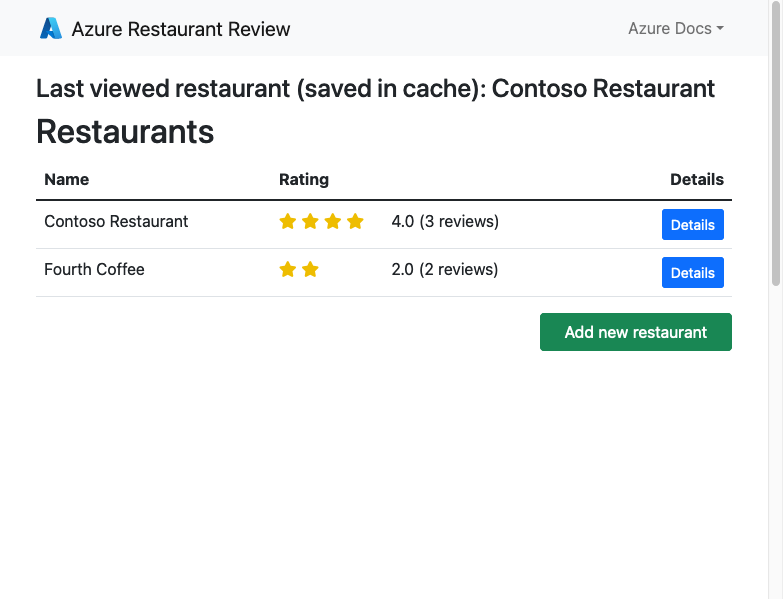This is an image of a website named "Azure Restaurant Review," featuring a logo with the letter 'A'. The 'A' is dark blue on the left and transitions to a lighter blue, like teal or turquoise, on the right. The interface displays a gray bar labeled “Azure Docs” with a drop-down arrow next to it. Just below, there are options titled "Last Viewed Restaurant," "Save and Cache," and "Consoso Restaurant." Further down, a prominent black heading states "Restaurants."

Under the heading, the site lists restaurant categories such as "Name," "Rating," and "Details." The first restaurant listed is "Consoso Restaurant," which has a four-star rating based on three reviews. Accompanying the review is a blue button labeled "Details" in white text. Below that, "Fourth Coffee" is listed with a two-star rating from two reviews, accompanied by the same blue "Details" button.

At the bottom of the list is a larger green bar labeled "Add New Restaurant," which can be clicked to add another restaurant for review.